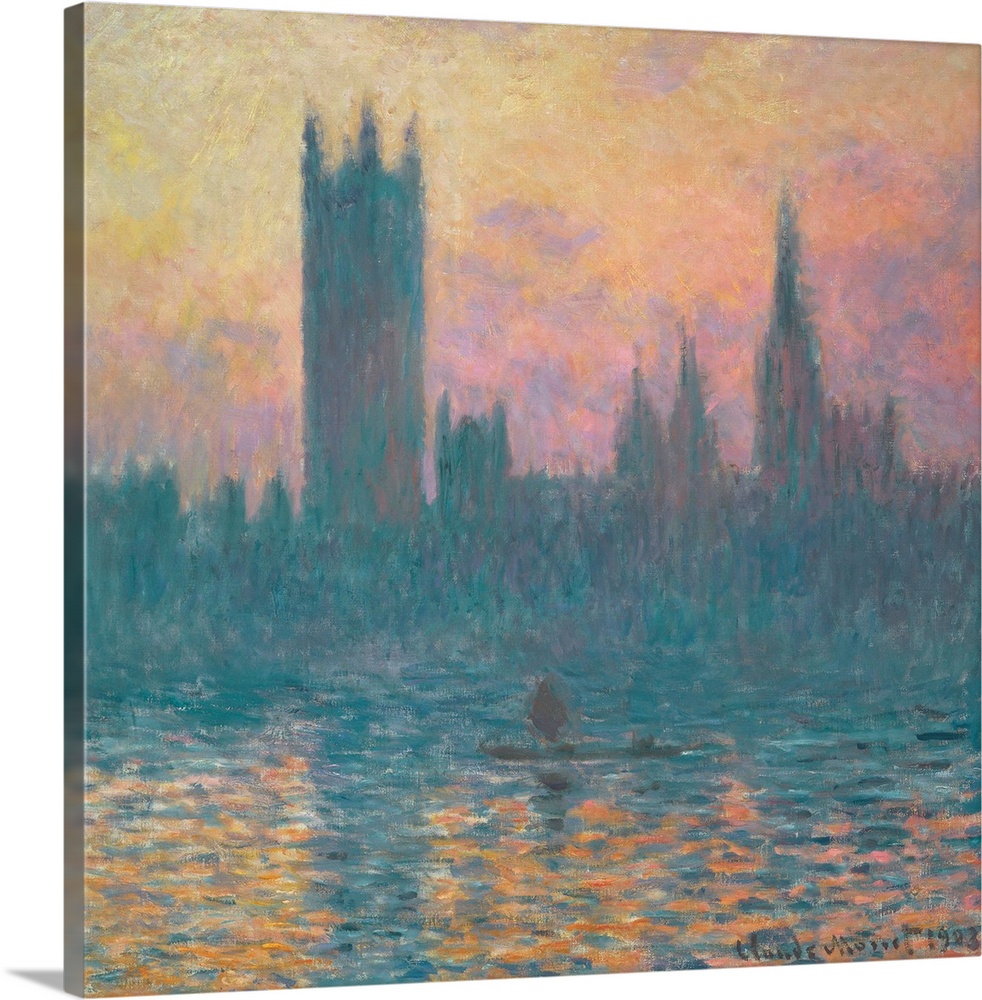The image is of a square painting that appears three-dimensional on the screen, casting a small shadow behind it due to the white background. The artwork itself is an abstract, Impressionist-inspired cityscape, reminiscent of Monet's style. The painting features varying heights of towers, with one significantly larger tower looming on the left. They are situated along what appears to be the River Thames, reflected in the colorful water below. The river is accented with a small boat traversing through the scene.

The scene depicted is either at dawn or sunset, with the sky transitioning from purplish hues at the bottom to radiant reds, oranges, and yellows at the top. This gradient of colors reflects beautifully in the water, creating an impression of sunlight dancing on the river's surface. The painting is rendered in oil, capturing the essence of the towers and their reflections with blends of purples, reds, oranges, and blues. Although a signature is visible at the bottom right of the painting, the name and the date, possibly 1903 or 1983, remain indiscernible.

Overall, this beautiful abstract piece evokes the impressionistic charm of a cityscape at either the break or close of day, with an exquisite interplay of colors reflecting city towers and a small rowboat on a serene river.